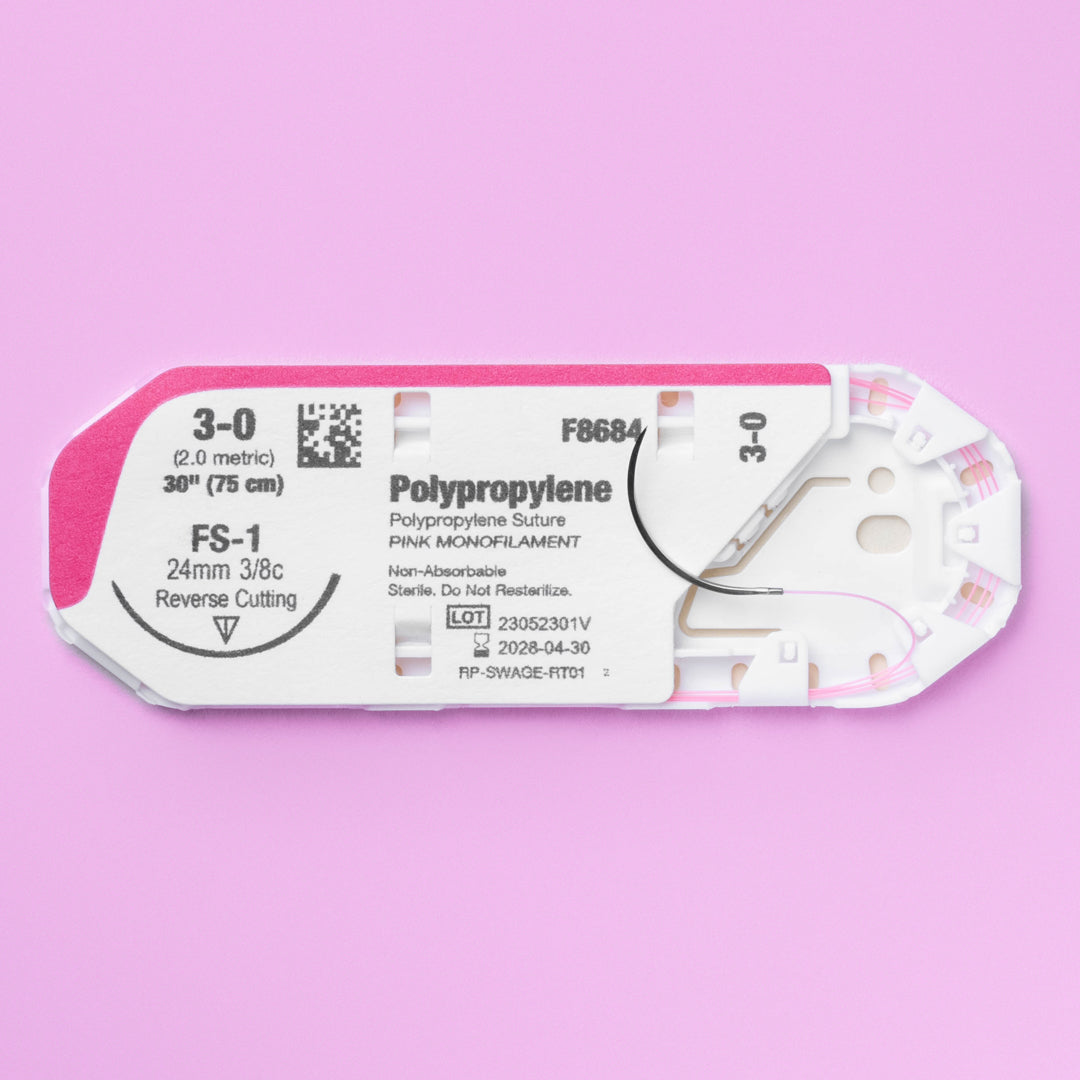The image depicts a close-up photograph of a rectangular medical device placed centrally against a pink background. The rectangular object, which appears to be a package for surgical sutures, is white with various texts printed on it. Dominating the center is the bold text "Polypropylene," with "Polypropylene suture" and "pink monofilament" noted below in smaller text. Other significant information includes "2.0 metric, 30 inches (75 centimeters), FS1, 24mm, 3/8C, reverse cutting." A number "30" is marked at the top and on the right side, with an arc-shaped design leading to a pink filament on the outer edge. Additionally, there is a QR code on the left, and toward the bottom, warnings such as "non-abrasive, sterile, do not re-sterilize" are indicated. A lot number "RP-SWHEE-RT01" and an expiration date "2026-04-30" are also printed on the package, ensuring its regulatory compliance. The device is designed for hospital use, specifically for surgical stitches, with careful detailing of its non-absorbable, hookless characteristic aiding in medical procedures.